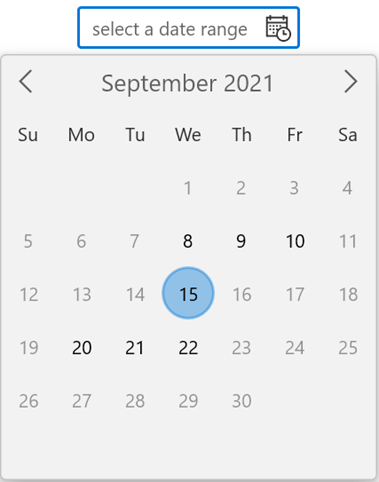The image displays a section of a website featuring a calendar interface. At the top, set against a white background, there is a bright medium blue border enclosing the phrase “select a date range,” which is written entirely in lowercase letters. Complementing this, small graphical icons of a calendar and a clock are positioned towards the top and bottom right sides respectively.

The main calendar section below this prompt rests on a light gray background. Prominently displayed at the top, the navigation arrows on the left and right allow users to cycle through months, while the center text denotes "September 2021." Directly underneath, the days of the week are succinctly represented by two-letter abbreviations with capitalized first letters: SU (Sunday), MO (Monday), TU (Tuesday), WE (Wednesday), TH (Thursday), FR (Friday), and SA (Saturday).

Specifically noted is the layout of the dates within this calendar: September begins on a Wednesday (the 1st) and extends, row by row, until Thursday the 30th. An additional detail highlights the 15th of September, which is distinctly marked by a blue circle around the number, evidently indicating a significant selection or event on that day.